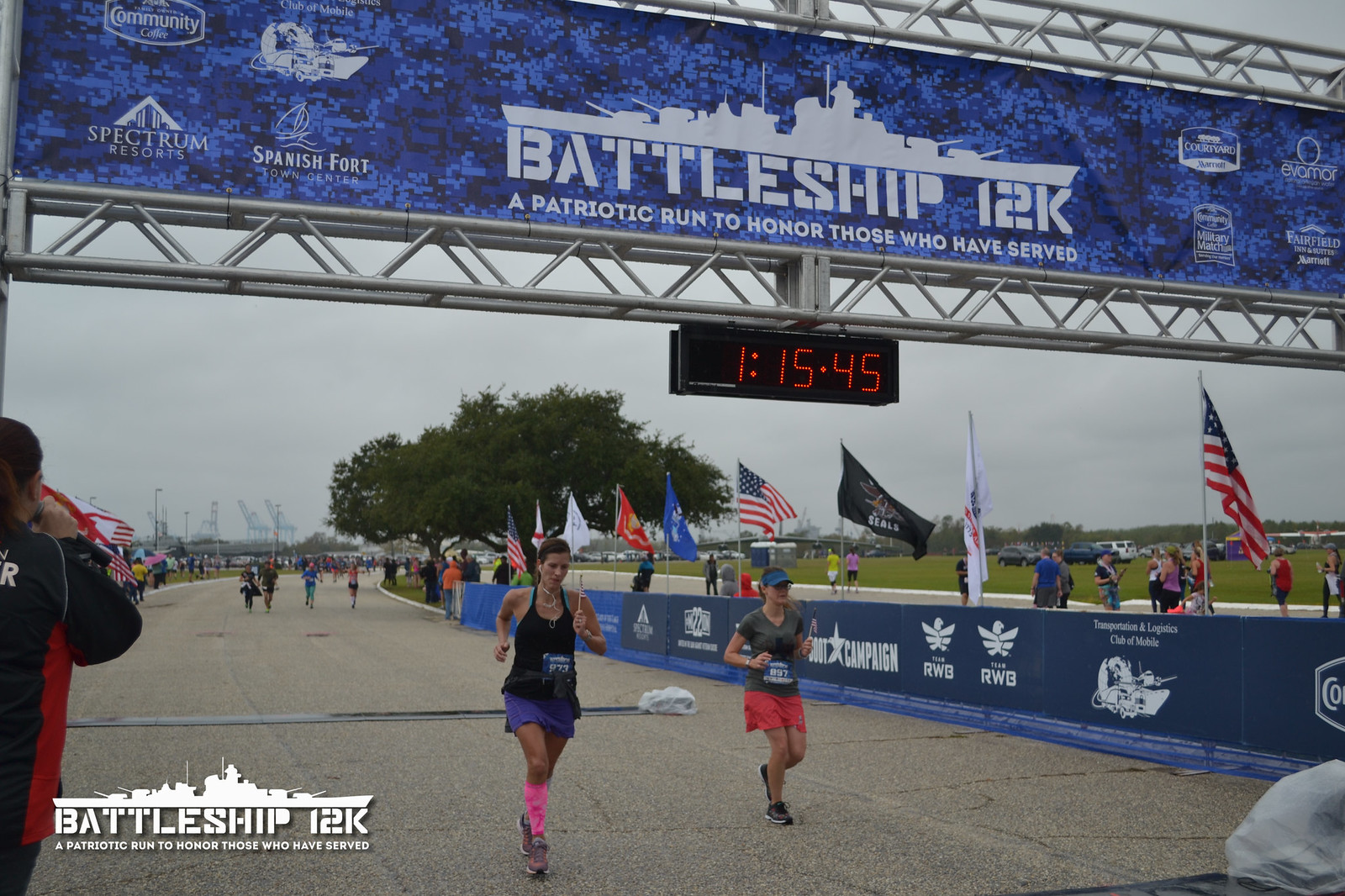The photograph captures the dramatic finish of a foot race, the Battleship 12K, prominently displayed on a blue banner above the finish line. The banner reads, "Battleship 12K, a patriotic run to honor those who have served," flanked by logos of sponsoring organizations such as Spectrum Resorts and Community Coffee. Below the banner and supported by metal archway bars, a digital clock shows a time of 1:15:45. Two women are crossing the finish line, the leading woman donning pink socks, a black shirt, and blue shorts. The setting includes a flat, paved race route adorned with numerous American and military flags lining the sides. Additional participants can be seen making their way towards the finish, encapsulating the spirit and dedication of the event. On the bottom left corner of the image, there's another emblem showcasing a battleship, reinforcing the race's theme and purpose.